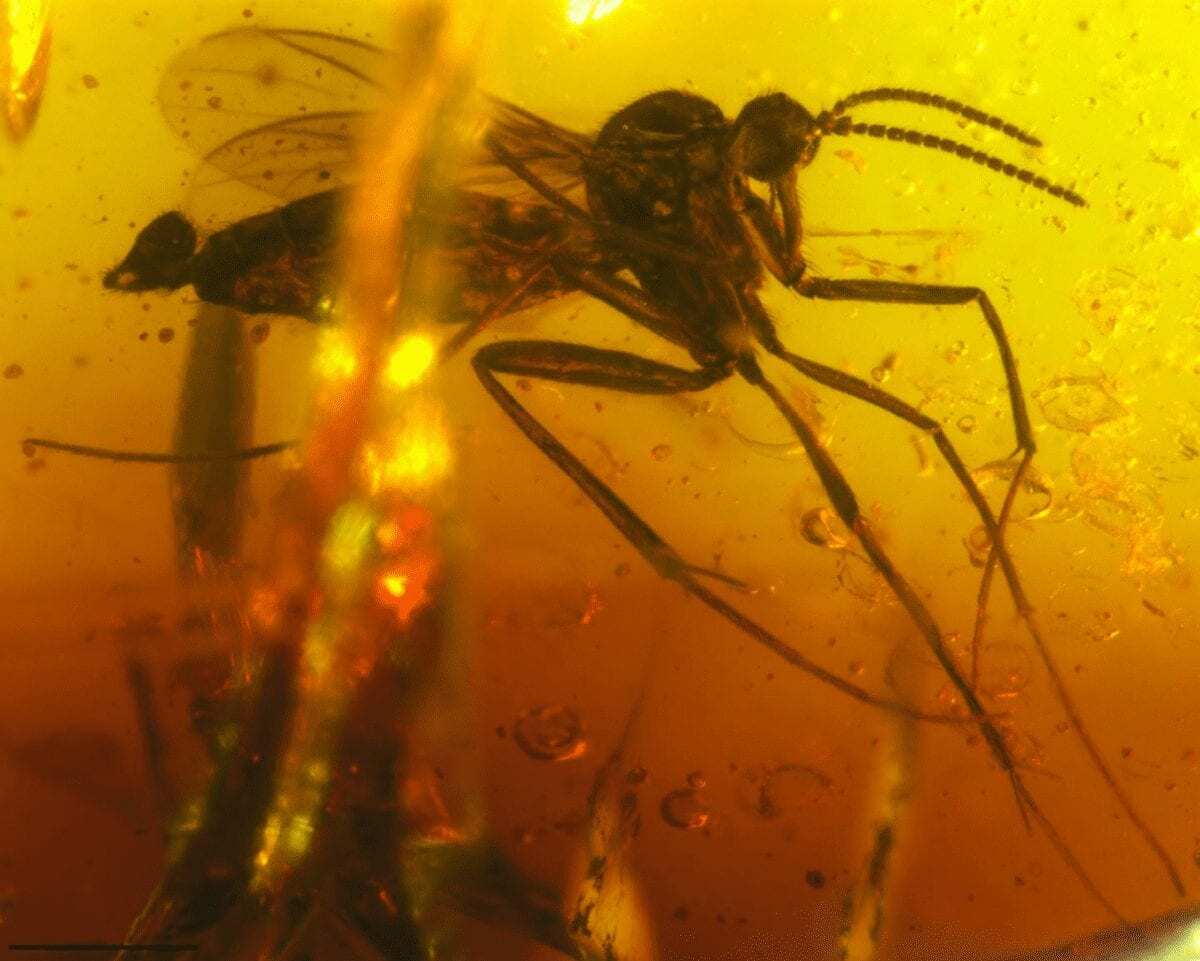This is an extremely close-up image of a dark brown mosquito-like insect, seemingly trapped in a chunk of amber, reminiscent of scenes from Jurassic Park. Its fine details are clearly visible, including the vein-like lines and brown spots in its large, transparent wings. The antennae are distinct, appearing as little spotted segments connected together. The insect's long, slender legs are prominently visible. The amber encasing it transitions from a yellow-gold hue at the top to an orange-red at the bottom, with a particularly bright spot of vivid yellow and red on the left side. The body of the insect is long and cylindrical, and it's surrounded by what look like drips of honey or sugar, enhancing the impression that it's frozen in time in this vibrant, colored substance.